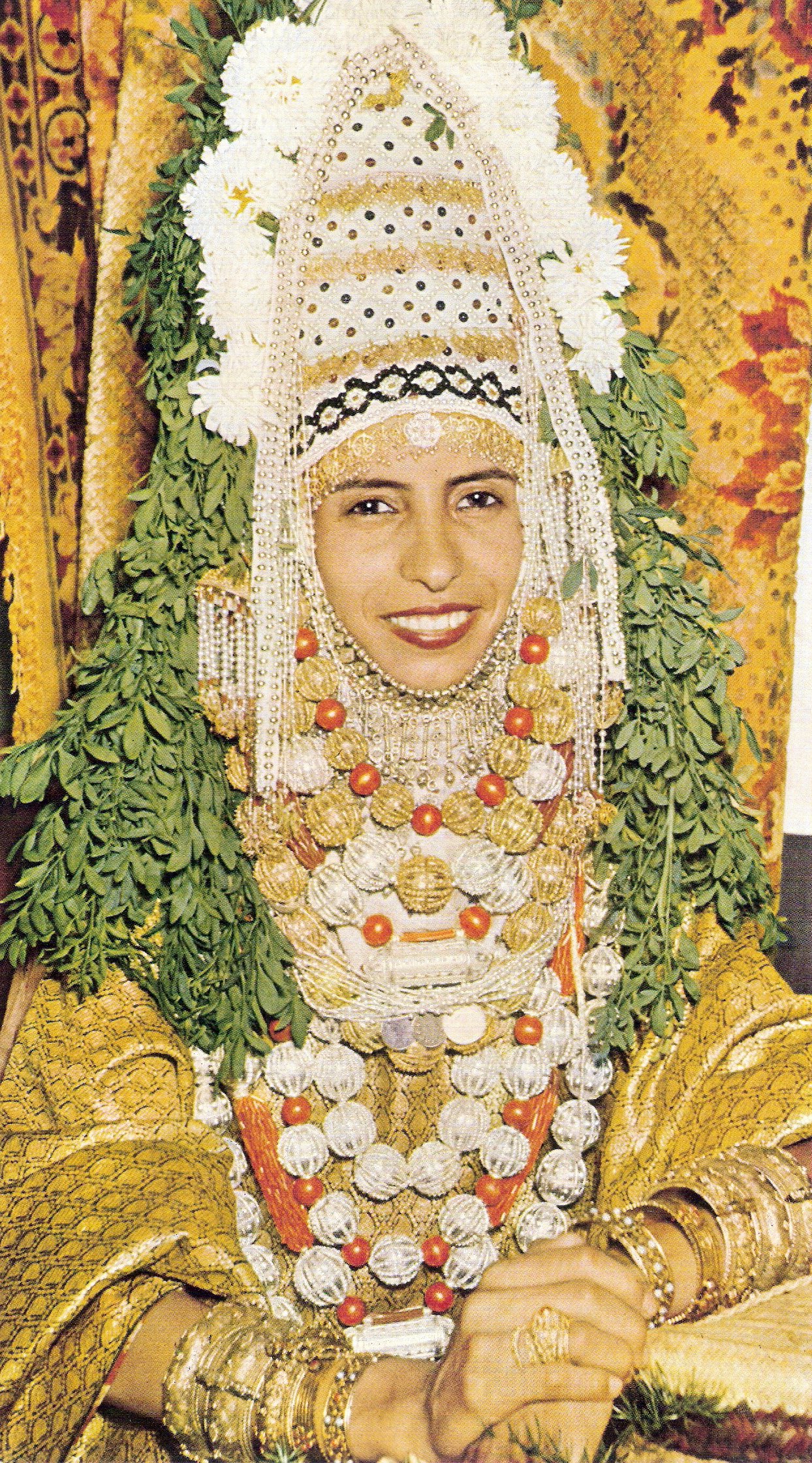In this detailed photograph, a woman is adorned in a striking traditional tribal outfit, suggesting a rich cultural heritage. The centerpiece of her ensemble is an elaborate cylindrical headdress, predominantly white with intricate beading and adorned with white flowers and small green leaves attached to the sides. The headdress frames her face, which is accentuated by red lipstick and a warm smile aimed at the camera.

Her attire further includes a sumptuous gold robe with a subtle black diamond pattern, exuding an air of opulence. This is complemented by a series of multi-colored necklaces featuring alternating silver and red beads, cascading across her chest. Additionally, she flaunts numerous gold bracelets that adorn her forearms, adding to the regal appearance.

The background of the image features green foliage, likely leaves, contributing a natural texture and contrast against the muted hues of the photograph, indicating it might be an older image. Tapestries with scarcely detailed patterns hang behind her, further enriching the cultural context of the scene.

Only her face, hands, and parts of her forearms are visible, the rest of her form ensconced in this magnificent regalia. The overall color scheme and the intricate detailing of her outfit reflect a deep cultural significance, preserved in this captivating photograph.